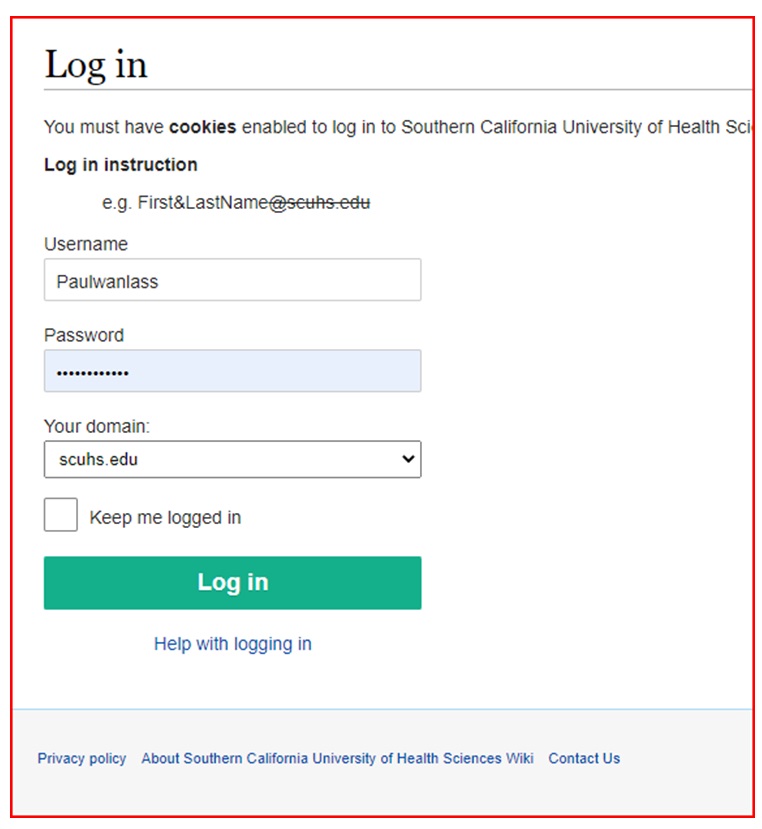A detailed screenshot of a login screen for the Southern California University of Health (SCUH) is depicted, possibly referring to Southern California Institute (SCI). The entire screenshot is bordered by a thin red line, with a clean white background inside. Positioned at the top left corner are the big, bold black letters that spell "Login," followed by a thin gray dividing line beneath it.

Underneath the header, a message states, "You must have cookies enabled to log in to Southern California University of Health SCI," although the message is partially cut off. Further down, there are login instructions, which read "E.G., for example, first&last name@SCUHS.edu." Notably, this example email address has a strikethrough applied, specifically on the second half.

The form fields are detailed as follows: In the username field, the text "Paul WANLASS" is entered. The adjacent password field contains masked characters represented by asterisks for security. Below these fields, the domain "SCHUS.edu" is indicated. Additional interface elements include a checkbox labeled "Keep me logged in," a prominent green "Log In" button, and a "Help with logging in" option likely meant to assist users experiencing login issues.